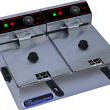The image depicts an extremely small and low-resolution color photo of a piece of machinery, set against a white background. The machinery is metal, predominantly powder-coated in grey, and the image is taken at a slight diagonal with the back of the object slanting upwards from left to right. The top of the device features two rectangular flaps with slight lips extending towards the viewer. Along the upper portion of the machinery, there's a black plastic strip that seems to function as a control panel or readout, complete with indicator lights and knobs. This control panel repeats a pattern of a green LED followed by a red LED, and a circular dial on both the left and right sides. Each flap on the top has two black dots that appear to be knobs and possibly handles or compartments below them. Despite the poor image quality, it appears to be some sort of electronic appliance, possibly a countertop kitchen device or machinery with pressing capabilities, although the exact function is indistinct due to the tight cropping and low resolution.